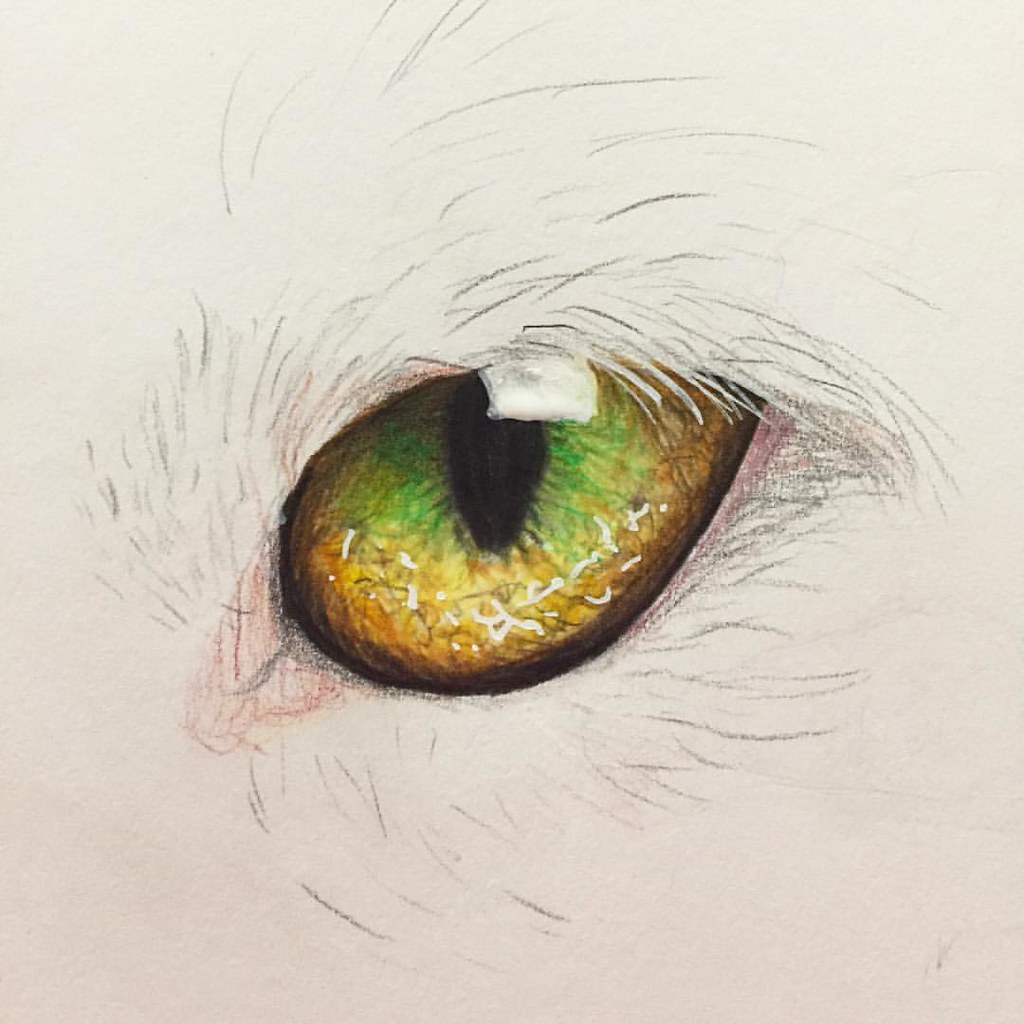This is a detailed charcoal drawing depicting a close-up of an animal's eye, likely a cat's, inferred from the distinct vertical pupil. The illustration lacks additional features that could confirm the animal's identity, focusing entirely on the eye itself. Charcoal streaks radiate around the eye, suggesting the presence of fur. The intricate details of the eye's coloring are meticulously rendered: the outer rim is a deep black, transitioning towards the pupil with an amber-brown hue embellished with white flecks, simulating corneal reflections. Closer to the vertical pupil, shades of lighter yellow and green become apparent. The top portion of the eye contains an area left white, possibly indicating a deliberate reflection or an unfinished aspect of the composition.